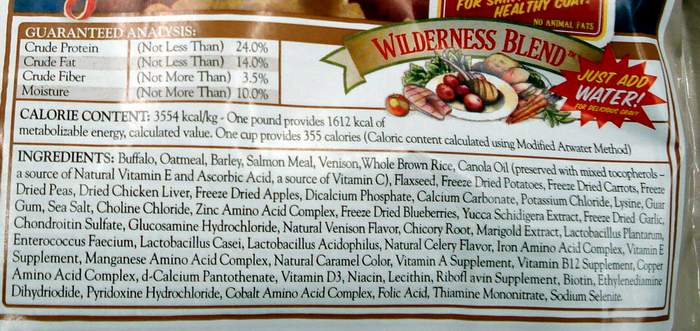This image showcases the back of a food product packaging, likely for animal food, given the specific nutrients listed. At the top of the white packaging with a dark brown border, there's a pale green banner featuring the bold red text, "Wilderness Blend." To the right, a prominent starburst declares "Just Add Water." Below, a whimsical cartoon-styled illustration displays a plate surrounded by various foods like carrots, potatoes, lettuce, and ham, with tomatoes on the plate.

The left side of the packaging details the "Guaranteed Analysis," listing crude protein at a minimum of 24%, crude fat at a minimum of 14%, crude fiber at a maximum of 3.5%, and moisture at a maximum of 10%. The calorie content is stated as 3,554 calories per kilogram, with one pound providing 6,012 calories of metabolizable energy. Additionally, one cup of the product offers 355 calories, calculated using the modified Atwater method.

Below this analysis, the ingredients are listed, including buffalo, oatmeal, barley, salmon meal, venison, whole brown rice, and canola oil. The light source, presumably from an overhead kitchen light, appears to illuminate the package from the top left.